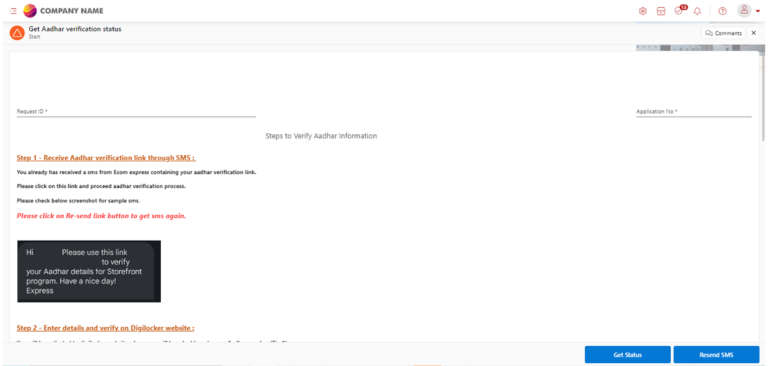Screenshot Description:

The image is a screenshot of a web page dedicated to AADHAR verification, likely from EcomExpress's website or a related service portal. The page is targeted towards guiding users through the process of verifying their AADHAR information for a storefront program.

- **Title and Steps**: 
   - At the top, the page has a title, "Company Name - Get AADHAR Verification Status" followed by a subheading, "Steps to Verify AADHAR Information".
   
- **Step One Explanation**:
   - The first step instructs users to "Receive AADHAR Verification Link Through SMS." It goes on to explain that users should have received an SMS from EcomExpress containing the necessary link. The instructions encourage users to click on this link to proceed with the AADHAR verification process. There is also a reminder to check a previous screenshot for sample use, and a "Resend Link" button for those who need the SMS to be sent again.
   
- **Black Box Description**:
   - Below this, there is a black box containing white text that says, "Hi. Please use this link to verify your AADHAR details for the storefront program. Have a nice day, EcomExpress."
   
- **Step Two Indication**:
   - The second step is partially visible and instructs users to "Enter Details and Verify on DigiLocker Website." The instructions cut off beneath this point.

- **Additional Information**:
   - The top left corner of the screenshot displays "Comments" and "Application Number".
   - At the bottom right corner of the image, there are two buttons labeled "Get Status" and "Resend SMS," each written in white lettering inside dark blue rectangles.

This screenshot does not show any people and is primarily focused on guiding users through the AADHAR verification process via detailed text instructions.